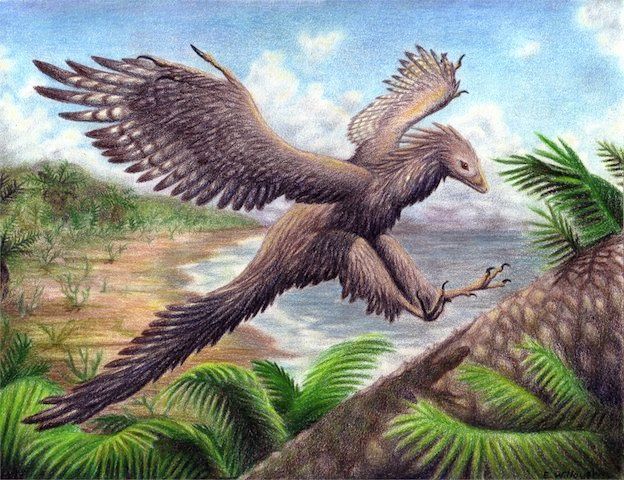This is a digital drawing depicting an ancient, predatory bird in mid-flight, preparing to land on a tree surrounded by lush foliage. The bird, which features brown wings adorned with white stripes, a sharp triangular face, and a tail reminiscent of a squirrel, appears reminiscent of a creature from the dinosaur era. Its sharp talons are extended forward, ready to grasp the shaft of the tree, which stands amidst an area filled with indistinct but dense green-brown foliage, possibly ferns and palm trees. The background showcases a serene, bluish-black body of water—likely a lagoon or sea—on the right, bordered by an orangish-brown shore that stretches from the foreground's left to the bottom right. Above, a bright blue sky dotted with fluffy white clouds completes the scene, giving it a dreamy, almost science-fictional atmosphere. The colors in the drawing are vibrant, emphasizing the contrast between the bird, the landscape, and the sky.